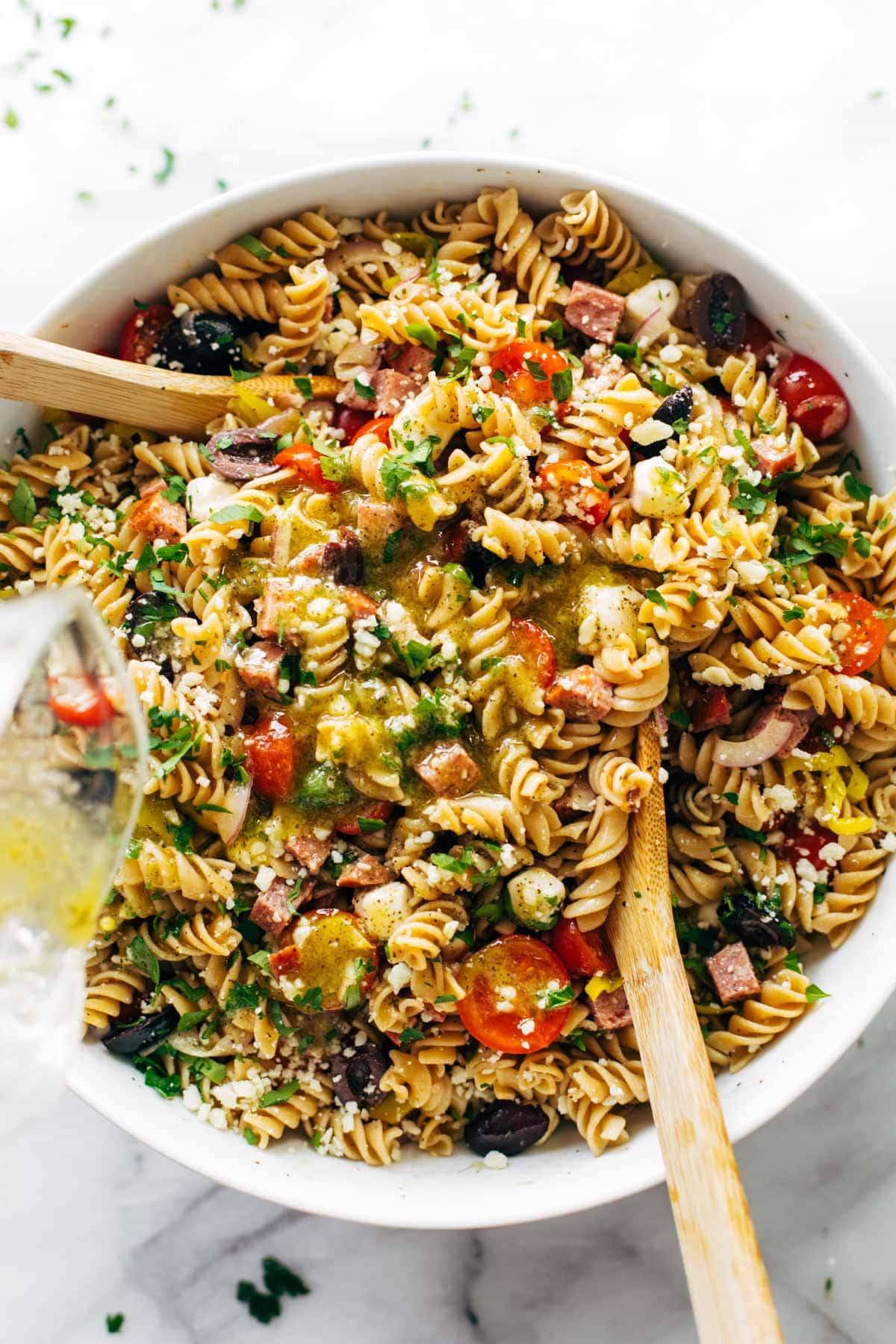This photograph features a vibrant and colorful pasta salad served in a pristine white bowl sitting on a white marble countertop. The star of the dish is a type of tri-spiral, rotelli, or rotini-shaped wheat pasta, complemented by halved cherry tomatoes, adding a burst of red to the ensemble. Mixed throughout are sliced black olives, chunks of ham, and a variety of possibly diced green leafy vegetables like parsley or chives, sprinkled generously. The salad appears to be dressed in a delightful oil-based dressing that gives it an orangish, golden-green hue, with hints of parmesan or feta cheese adding a savory touch. Populated with additional ingredients such as chickpeas and yellow peppers, the dish is both visually appealing and presumably nutritious. Two large wooden serving spoons are elegantly placed within the bowl, ready for serving this abundant and delicious pasta salad.